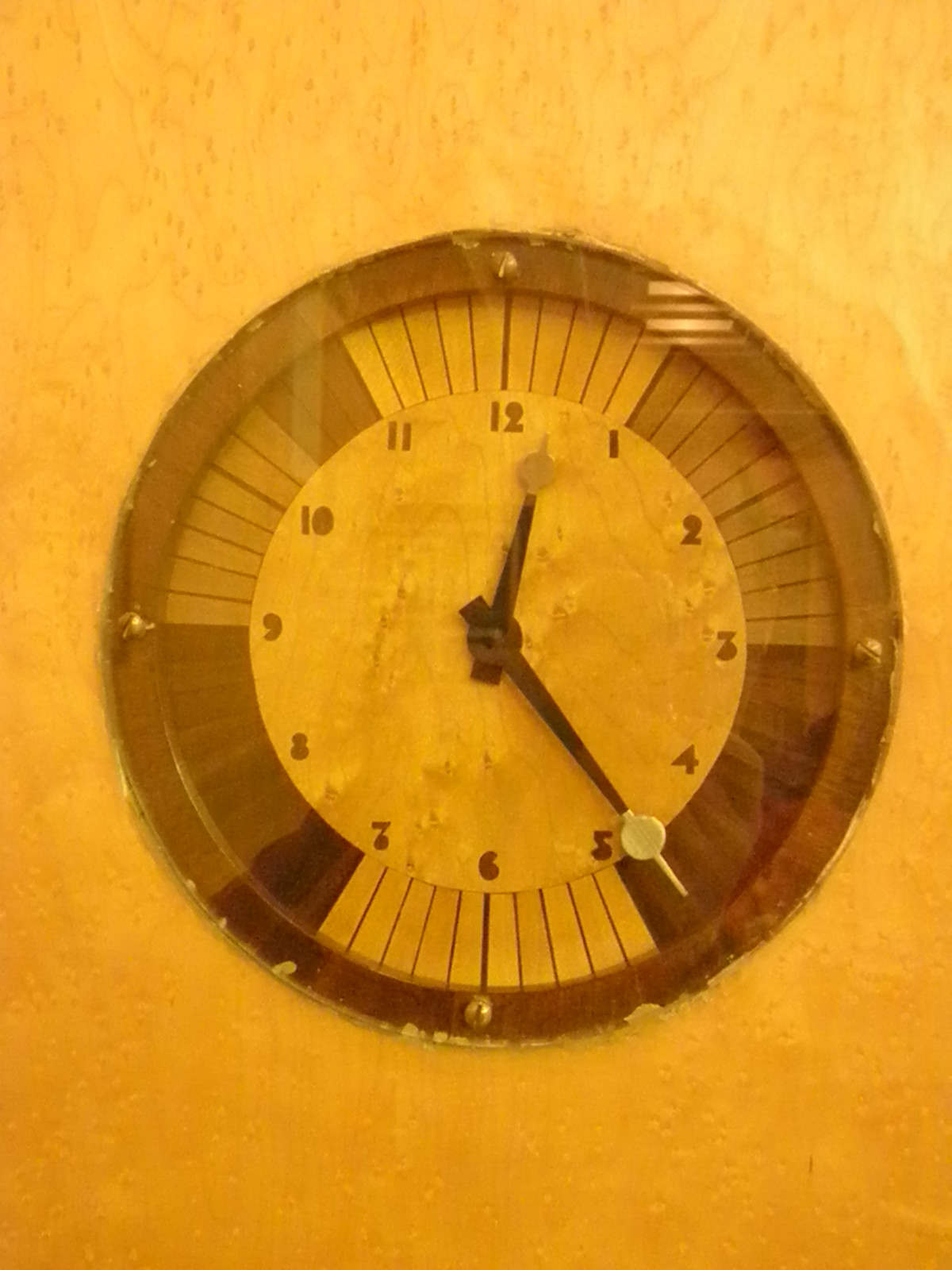This photograph showcases a striking round clock mounted on a yellowish-orange wall that transitions from a lighter hue at the top to a darker shade at the bottom, resembling plywood. The clock's circumference is adorned with several small pieces of wood glued together in a circular pattern, enhancing its rustic appearance. Secured with four screws—one each above the 12, below the 6, to the left of the 9, and to the right of the 3—the clock features a brown face with numbers in a darker brown shade. 

The outer border of the clock displays sections of varying colors: a yellow segment above the 11 and 1, a greyish tint between 1 and 3, a reddish-brown area between 3 and 5, another yellow portion between 5 and 7, a darker brown section from 7 to 9, and a lighter grey segment from 9 to 10. The black hour hand is just past the 12, while the minute hand, featuring a distinct round white tip with a sharp point, is positioned just before the 5. The overall yellowish tint in the photograph is likely due to the harmonious coloring of both the clock and the wall.